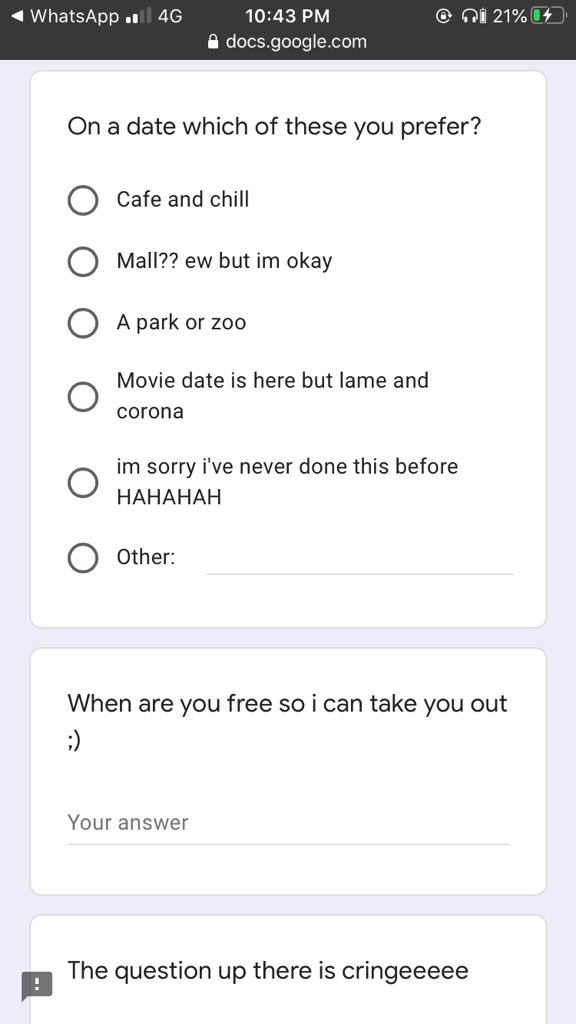Here is a more refined and detailed version of the given caption:

---

This screenshot captures a WhatsApp conversation interface on a smartphone. At the top, a back arrow is visible along with the text "WhatsApp." To the right, the status bar displays "4G" signal strength, the time "10:43 PM," a padlock icon indicating a secure connection to "docs.google.com," and icons for headphones and the battery level at 21%.

Below the status bar, a light purple-bordered box contains a survey question in a white background: "On a date, which of these do you prefer?" followed by selectable bubbles for response options. These options include:

1. Cafe and chill.
2. Mall?? (you, but I'm okay).
3. Park or a zoo.
4. Movie date (lame and Corona).
5. I'm sorry, I've never done this before hahaha.
6. Other (with a line for entering a suggestion).

Beneath this survey, another question asks, "When are you free so I can take you out?" accompanied by a winking face emoji and a line for writing a response.

At the bottom, there's an exclamation point box next to the statement, "The question up there is cringy."

---

This detailed caption provides a clear and structured description of the content in the captured smartphone screenshot.